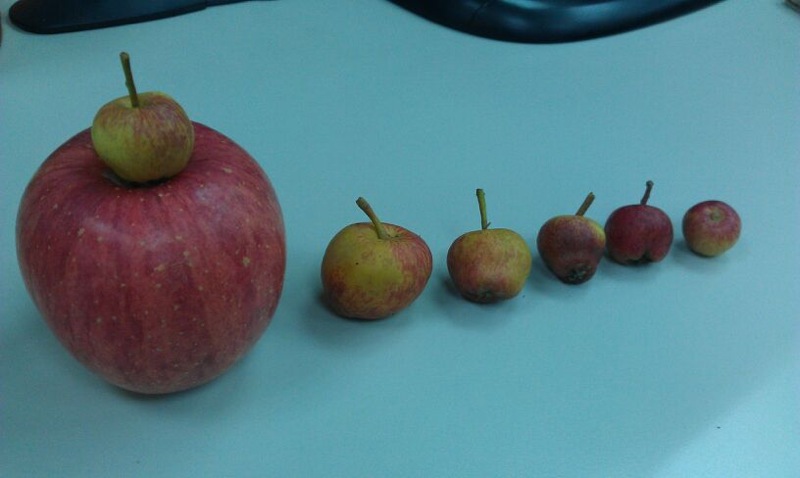In this intriguing image, six apples are meticulously arranged on a bright blue surface, creating a striking visual contrast. The apples are lined up from left to right, varying dramatically in size, color, and condition. The lineup starts with a very large, vibrant red apple, which interestingly has the smallest apple—mostly green with patches of brown and a hint of red, perched on top, accentuating the size disparity. This tiny apple, despite its diminutive stature, has a prominent stem jutting out.

Continuing along the row, the second apple mirrors the small one’s greenish hue with specks of reddish-brown, but it rests alone and is slightly larger. Each successive apple decreases in size and exhibits a blend of these color patterns to varying degrees. The third apple is similar in color to the second but is marginally smaller and features a straight stem. The fourth apple deviates slightly in shape, being more pear-like, and is mostly red with a crooked stem.

The fifth apple is notably all red and appears ripe and robust, with a straight-standing stem. Finally, the last and smallest apple is predominantly red with tinges of green and lacks a stem altogether. The bright blue background adds a vivid contrast, showcasing the apples' diverse hues and emphasizing their arrangement from largest to smallest. Additionally, a reflection on the blue surface suggests a glossy finish, and there's a faint glimpse of what could be pots or pans with a black handle in the corner, adding a subtle context to the setting.